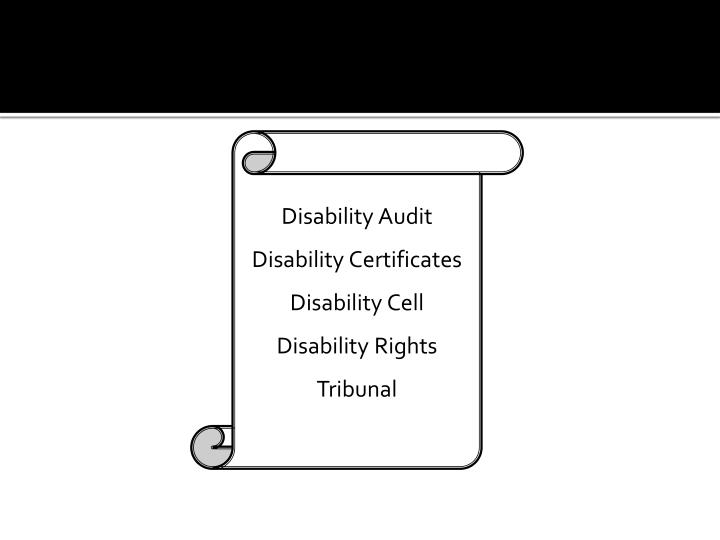The image features a white scroll, designed with shades of gray and outlined in black, set against a large black rectangular background. The scroll, which appears to be rolled up at the top, lists several terms in a combination of upper and lower case letters. The terms are presented in the following order: "Disability Audit," "Disability Certificates," "Disability Cell," "Disability Rights," and "Tribunal." The black font on the white scroll stands out clearly, but there is no additional information provided about the context or process related to the listed terms.